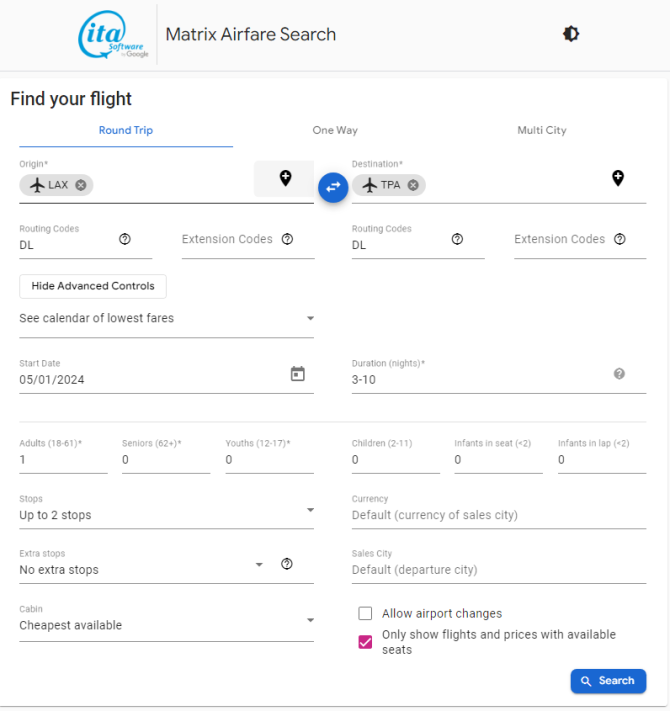The image depicts the homepage of an airfare search website titled "Matrix Airfare Search" powered by ITA Software, a subsidiary of Google. The top of the page features a toggle button to switch between light mode and night mode. In the upper left corner, a prominent section labeled "Find Your Flight" offers selection options for round-trip, one-way, or multi-city itineraries.

Below this, fields are provided for inputting origin and destination airports, which in this instance display "LAX" (Los Angeles International Airport) and "TPA" (Tampa International Airport) respectively. Additional boxes for routing and extension codes are available for both the departure and arrival flights. There is an option to hide advanced controls, as well as a link to view a calendar of the lowest fares.

The current search parameters include a start date of May 1, 2024, with a trip duration ranging between 3 to 10 nights. The form queries the number of travelers, split into categories such as adults, seniors, youths, children, infants in seats, and infants in laps, with one adult selected in this case. Travel options also cover up to two stops, no extra stops, and the cheapest available cabin.

Additional features include currency and city of sale options. A box labeled "Allow Airport Changes" is unchecked, whereas another option to "Only Show Flights and Prices with Available Seats" is selected. A search button is located at the bottom right-hand corner of the form for initiating the flight search.